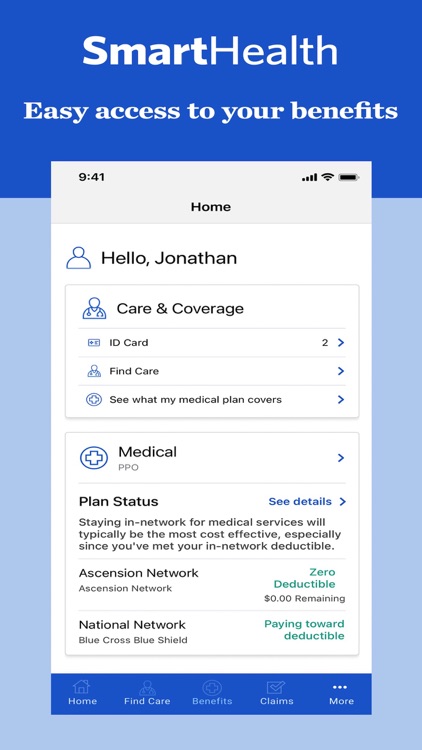This image captures a mobile screenshot of the SmartHealth app's home page. At the very top, "SmartHealth" is presented in large white font, followed by the phrase "Easy to access your benefits" in bold white lettering. The main focus of the screenshot shows the app's home page.

The app's interface is organized and user-friendly, starting with a gray header that centrally features the word "Home" in bold black letters. Just below this, the screen transitions to a clean white background. In the top left corner, there's a blue profile icon with the welcoming message, "Hello Jonathan," in large black letters to its right.

A prominently outlined gray box follows, labeled "Care and Coverage." Below this box, a vertical list of options allows users to easily navigate through different functionalities including "ID Card," "Find Care," and "See What My Medical Plan Covers."

Following this section, there's another large gray outlined box titled "Medical." Inside this box, the text "PPO" is displayed in small gray letters. The section provides further details about the user's plan status, with a "See Details" link in blue letters to the right. It also mentions the "Ascension Network," noting a "Free Deductible" or "Zero Deductible," and the "National Network," with a status update on "Paying Toward Deductible."

At the very bottom of the screenshot, a navigation bar lists essential app options such as "Home," "Find Care," "Benefits," "Claims," and "More," making it easy for users to access different areas of the app efficiently.